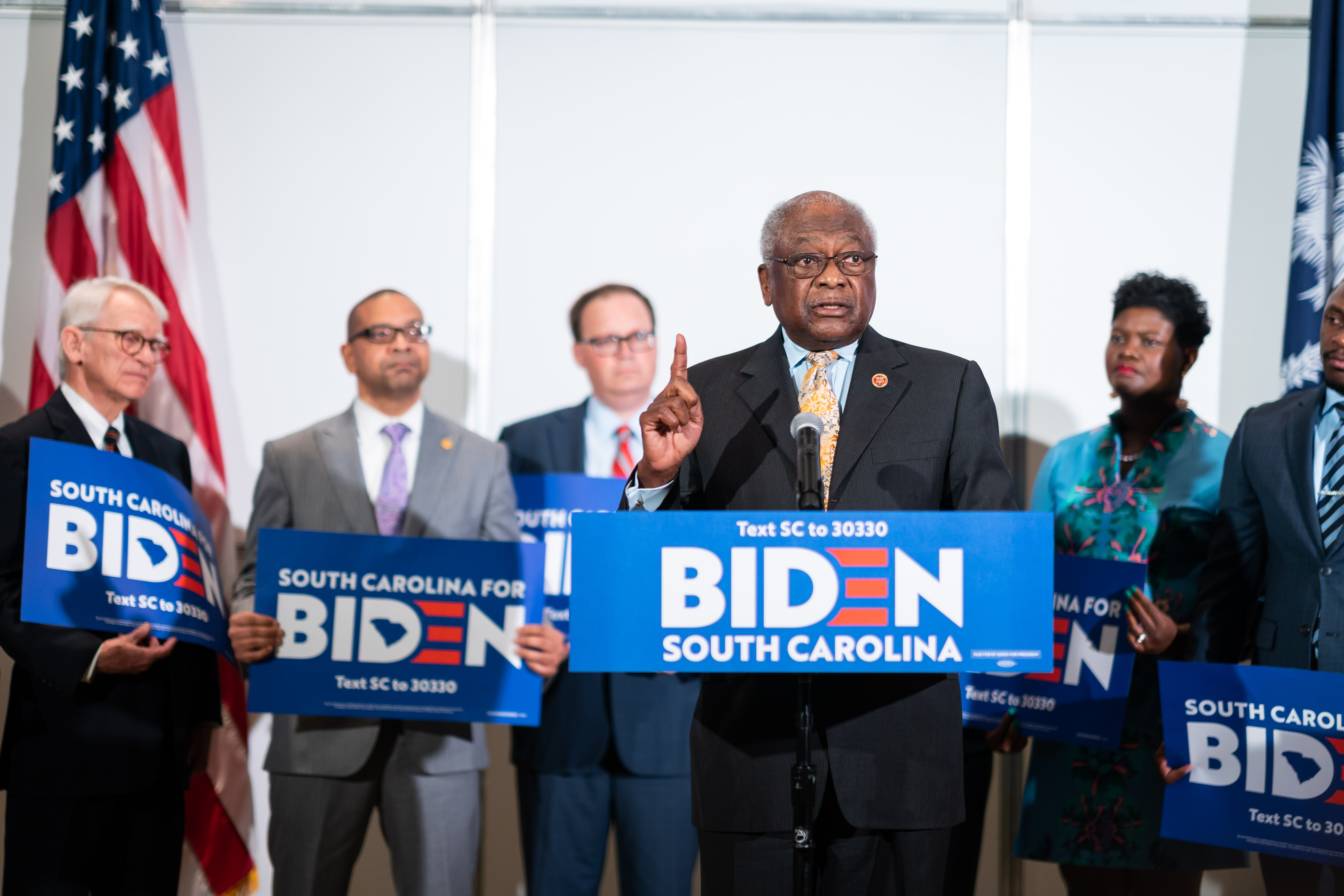This image captures a lively campaign rally for Joe Biden in South Carolina, featuring six people—five men and one woman—positioned in front of a backdrop with an American flag on the left and what appears to be the South Carolina state flag on the right. At the forefront is an African-American man with male pattern baldness and white hair, clad in a dark suit, a light blue shirt, and a yellow and gray patterned tie. He sports glasses and a bright red symbol on his lapel pin, standing at a podium with a blue sign that reads "Text SC to 30330 Biden, South Carolina," marked by a distinctive red 'E'. This gentleman, who is the focal point of the photo, is addressing the audience with a microphone, gesturing confidently with a single finger pointed upwards.

Behind him stand the rest of the attendees. To his left are three men, all in glasses, each holding "South Carolina for Biden" placards. A woman, appearing to be in her 40s, listens intently while also holding a Biden sign, positioned slightly to his right. Another younger gentleman stands further to the far right, close to the state flag, joining the others in support with his own placard. The overall scene strongly conveys the enthusiastic and united front of this group as they campaign for Biden in South Carolina.